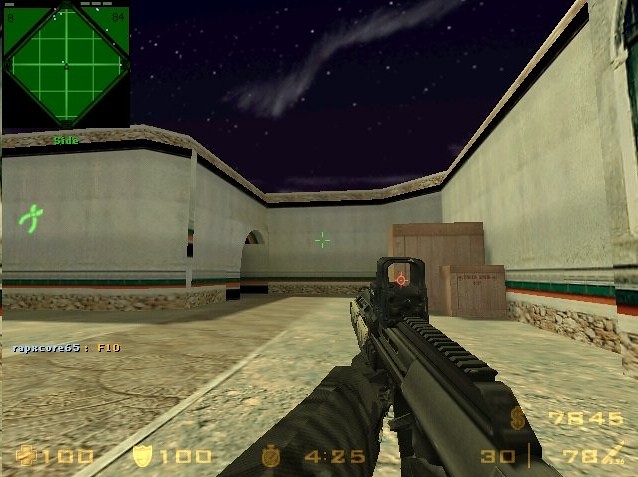In this nighttime scene from what appears to be the video game Counter-Strike, the sky is dotted with numerous stars and a single cloud. The top left corner of the screen features a green, diamond-shaped map overlay. Below this map, a green icon of pliers is displayed. Additionally, the player with the username "rapxcore65" is seen typing "F10" in the in-game chat. Along the bottom of the screen, orange text shows "100" next to a stamina or health indicator, with a stopwatch reading "425". In the bottom right corner, the player's money is displayed as "$7,845," and ammunition details reveal "30/70," indicating the gun is loaded with 30 bullets out of a possible 70. The player, in a first-person perspective, wields a green firearm equipped with a holographic scope, centered by a green crosshair. The setting features buildings constructed from white and tan concrete, surrounded by wooden crates.